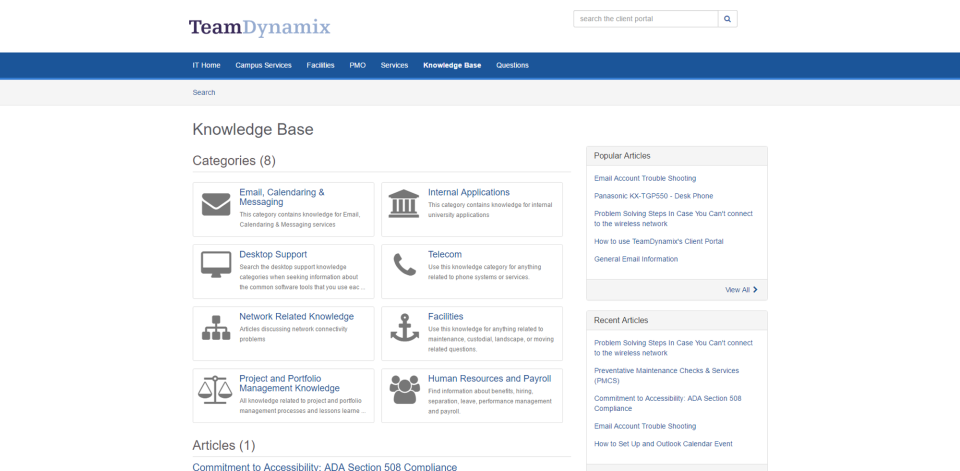At the top of the webpage, "Team Dynamics" is prominently displayed. Directly beneath this title, a blue rectangle spans the entire width of the page, containing text approximately two-thirds of the way across, though the text is too small to discern clearly. Below the blue rectangle, a gray rectangle features a "Search" bar. Beneath the search bar, the title "Knowledge Base" appears in bold black text, followed by "Categories" and the number "8".

The categories are displayed in two columns, each accompanied by small icons:

- **First Column:**
  1. Email, Calendaring, and Messaging
  2. Desk Support
  3. Network-related Knowledge
  4. Project and Portfolio Management Knowledge

- **Second Column:**
  1. Internal Applications
  2. Telecoms
  3. Facilities
  4. Human Resources and Payroll

To the right, a third column titled "Popular Articles" lists five articles in small blue text. Below this, a section titled "Recent Activities" also lists five recent activities in blue writing.

At the very bottom left of the page, an article titled "Commitment to Accessibility – ADA Section 508 Compliance" can be found.